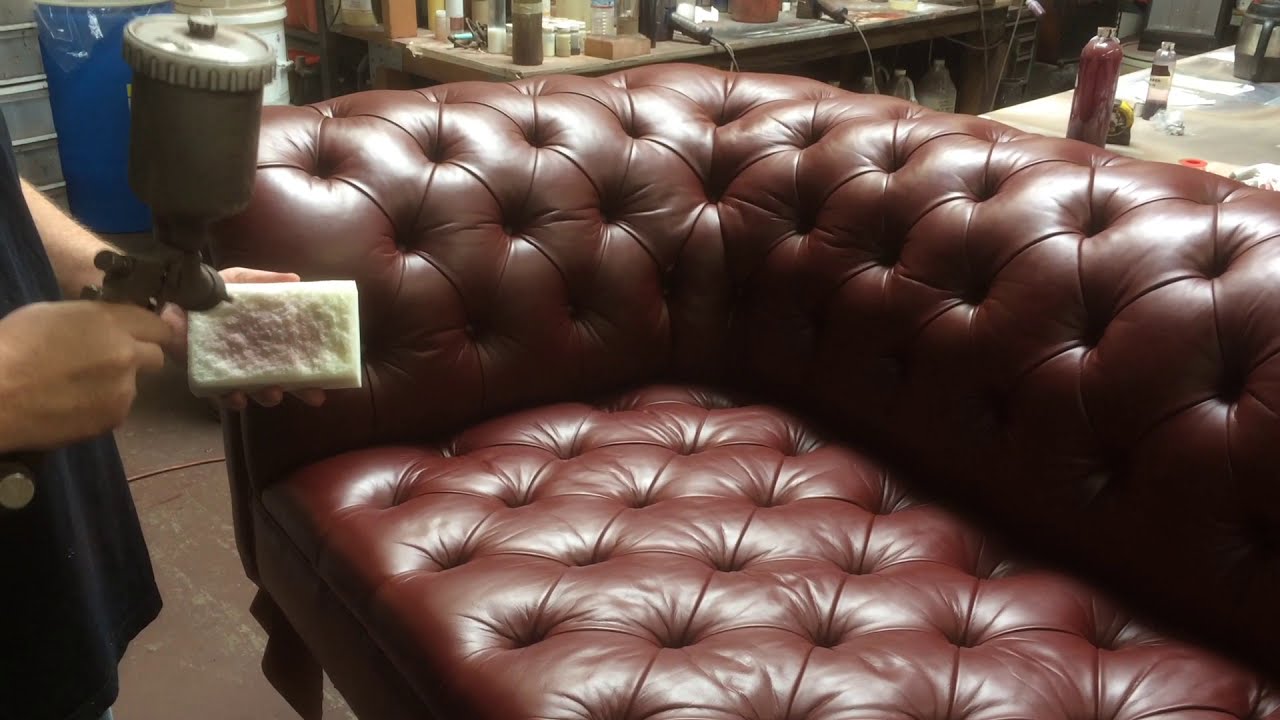The photograph depicts a woman in a workshop, engaged in restoring a Chesterfield-style, tufted leather couch. The maroon or brown-colored sofa features the characteristic deep button-tufted design with divots every six inches. Clad in a dark shirt and possibly an apron or smock, the woman is holding a sponge in her left hand and a spray gun-like tool in her right, dispensing a conditioning product onto the sponge, which shows traces of the sofa’s color. In the background, various tables laden with numerous bottles of different colored liquids and tools suggest an environment dedicated to furniture restoration.